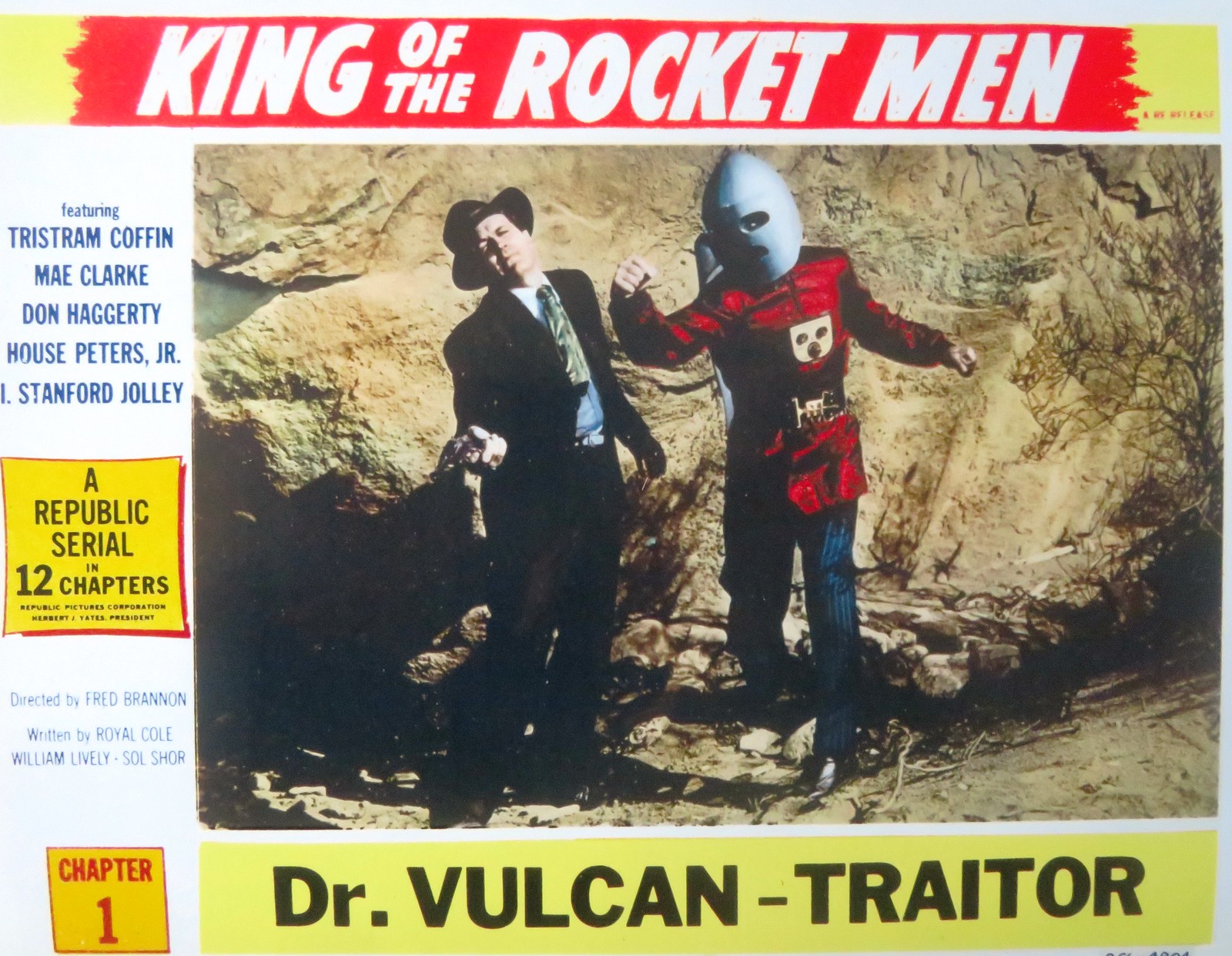This image is a detailed poster of an old sci-fi show. Dominating the top section is a red banner with bold white letters that read, "King of the Rocket Men." The left side of the poster lists the featured cast in blue letters: Tristram Coffin, Mae Clark, Don Haggerty, House Peters Jr., and I. Stanford Jolley. Below the banner, the poster depicts an action scene set against a rocky backdrop under a sunny sky. On the right, Rocket Man is seen in a dynamic pose, wearing a metallic helmet shaped like the top of a rocket, a red jacket reaching his mid-thigh, blue pinstripe pants, and black shoes. Rocket Man's mask has eye and mouth cutouts, and he's in the midst of throwing an uppercut punch with his right hand. His left arm extends to the side for balance. His opponent on the left, wearing a dark suit, a bluish collared shirt, and a green tie, has his head tilted back with his eyes closed, suggesting he has just been hit. He holds a gun loosely in his right hand, which is about to drop. A yellow square near the top reads, "A Republic Serial in 12 chapters," while another yellow banner at the bottom states, "Dr. Vulcan - Traitor" in red letters. At the very bottom left corner, a tiny red block displays "Chapter 1."